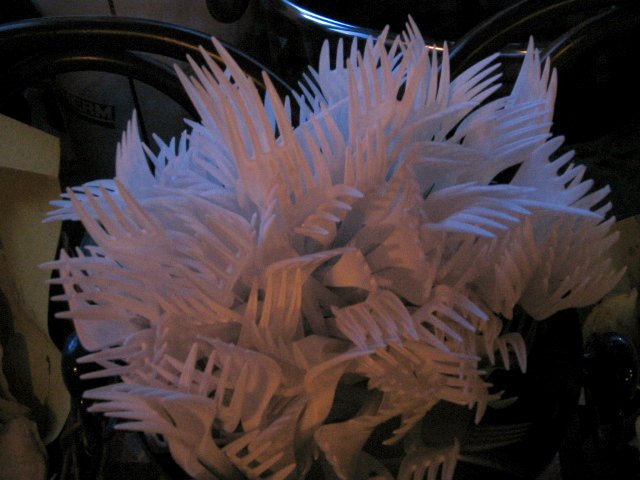The image is a close-up, landscape-oriented photograph focusing on a densely packed collection of roughly 40 white plastic forks, all with their tines facing upwards towards the camera. These forks are held together tightly, appearing somewhat entangled, in a black container resembling a large cup. The scene around the forks is cluttered; to the left, there is a piece of brown paper with its edges creased and sticking up, and nearby are yellow post-it notes, crumpled and slightly discolored under poor lighting. Thick black wiring is visible to the left and above the forks, with some lettering partially obscured by the wires and post-it notes. On the top right, a black handle and a small dial or knob can be seen, adding to the image's overall busy and grainy appearance.